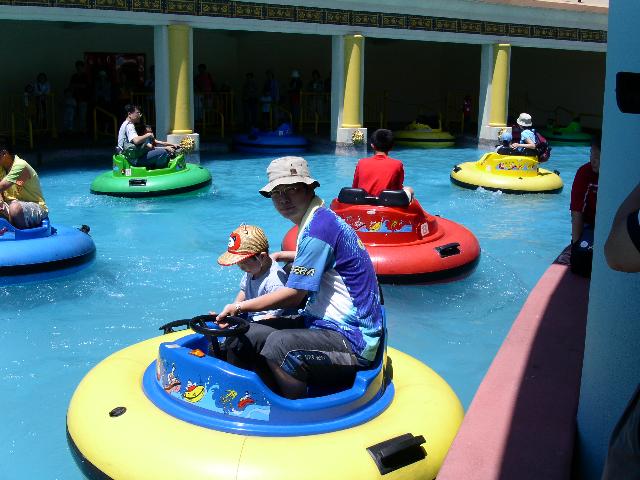The photograph captures a lively scene at a water park where families are enjoying a bumper boat ride in a clear, blue pool. The image foregrounds a man in a blue shirt and black shorts, accompanied by his young son in a gray shirt and brown baseball cap, both seated in a yellow bumper boat. The son is attempting to steer the boat with a black steering wheel while the father keeps a watchful eye. Surrounding them are four other colorful bumper boats – a blue one to the left piloted by a partially visible man in tan shorts and a yellow shirt; a red one just behind with an older boy wearing a red T-shirt; another yellow boat further back helmed by a woman with a brown hat and backpack; and a green boat at the left rear with a man and a young child aboard. Enclosing the area are three yellow pillars supporting a roof structure, adding to the sense of an amusement park environment.